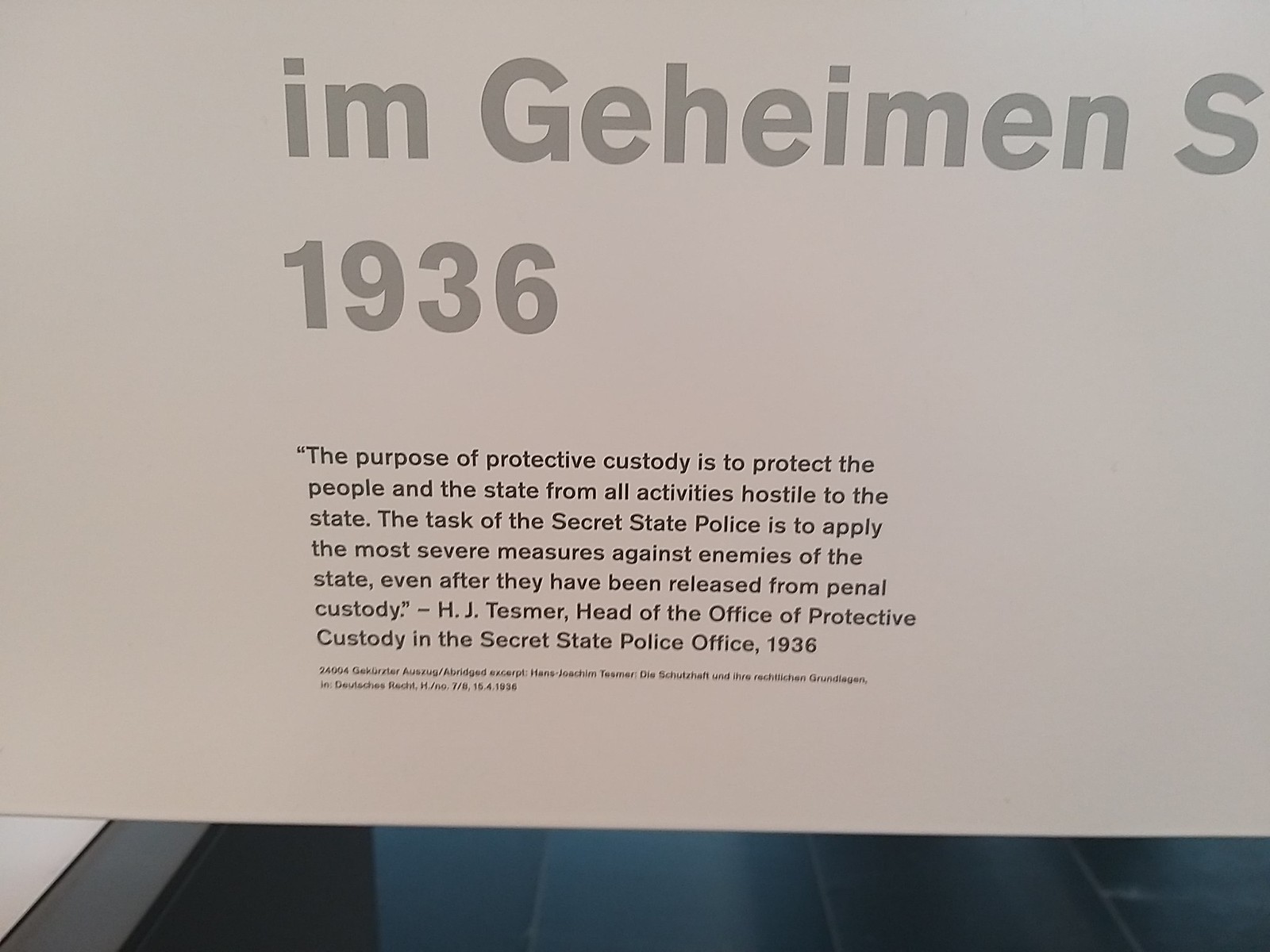The image features a rectangular sign measuring approximately six inches wide by four inches tall. Dominated by a light brown background, the sign has intricate details that stretch from the upper left-hand corner to the upper right-hand corner and extend down both sides, stopping about three-quarters of an inch from the bottom. 

The top center of the sign features lowercase brown text reading "i am," followed by a capitalized "G" and the name "Geheimen" spelled "G-E-H-E-I-M-E-N." A capital letter "S" is visible but cuts off as it extends out of frame. Below this, the year "1936" is prominently displayed in bold lettering. 

The central part of the sign contains a paragraph encased in quotation marks: "The purpose of protective custody is to protect the people and the state from all activities hostile to the state. The task of the Secret State Police is to apply the most severe measures against enemies of the state, even after they have been released from penal custody." This quote is attributed to "H. G. Tesmer, head of the Office of Protective Custody in the Secret State Police Office, 1936." Below this, there is some very small and unreadable text.

The bottom portion of the image shows a blue-tiled surface, suggesting the sign may be resting on a countertop or floor. On the left-hand side of the image, a fragment of a gray wall is visible. Overall, the sign appears to be informative, possibly historical in nature, relating to the activities of a police organization.